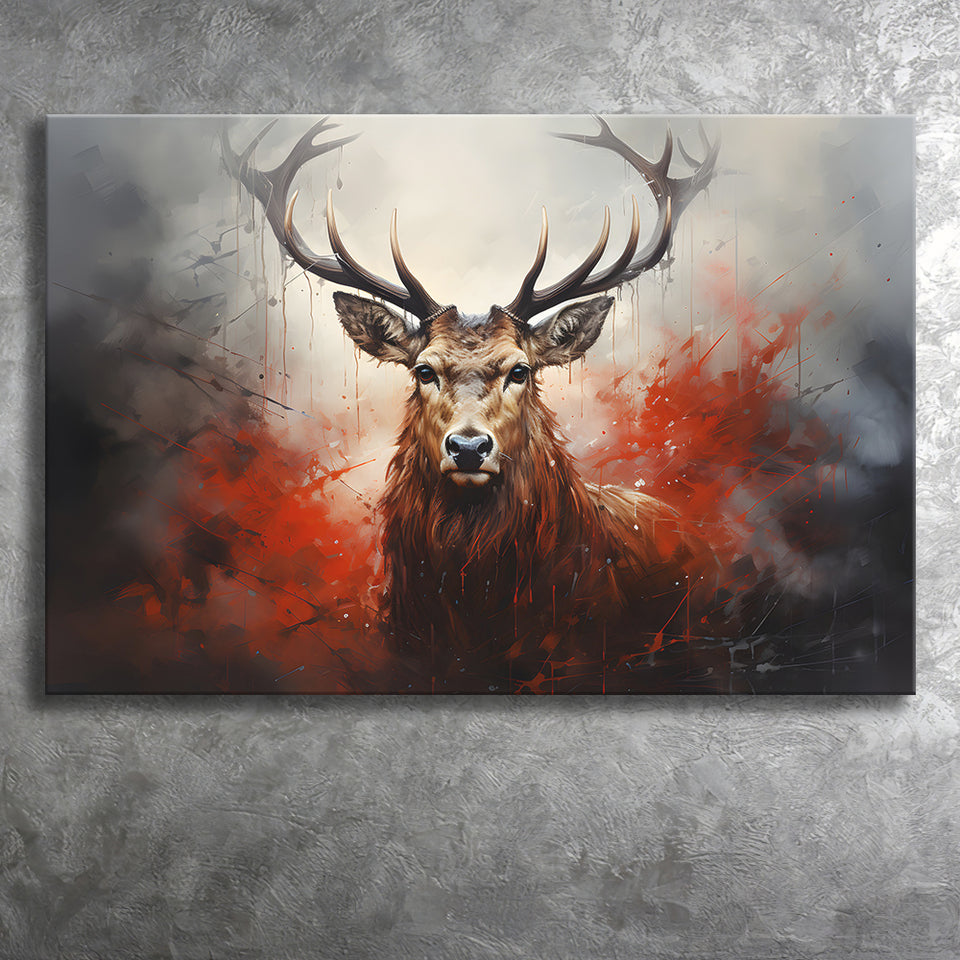The hyper-realistic painting depicts a magnificent deer with thick, textured fur, staring directly into the eyes of the viewer. Its large rack of antlers, from which velvet strips and paint drips seem to cascade, captures immediate attention. The deer, rendered in rich shades of brown, stands against an unframed canvas mounted on a textured grey wall. Surrounding the deer is an abstract, splattered design in black, red, and grey hues, which becomes increasingly smudged and diffused towards the canvas edges. This combination of hyper-realism in the deer's detail and the painted, more animated style of the background creates a captivating contrast that draws the observer deeply into the scene.